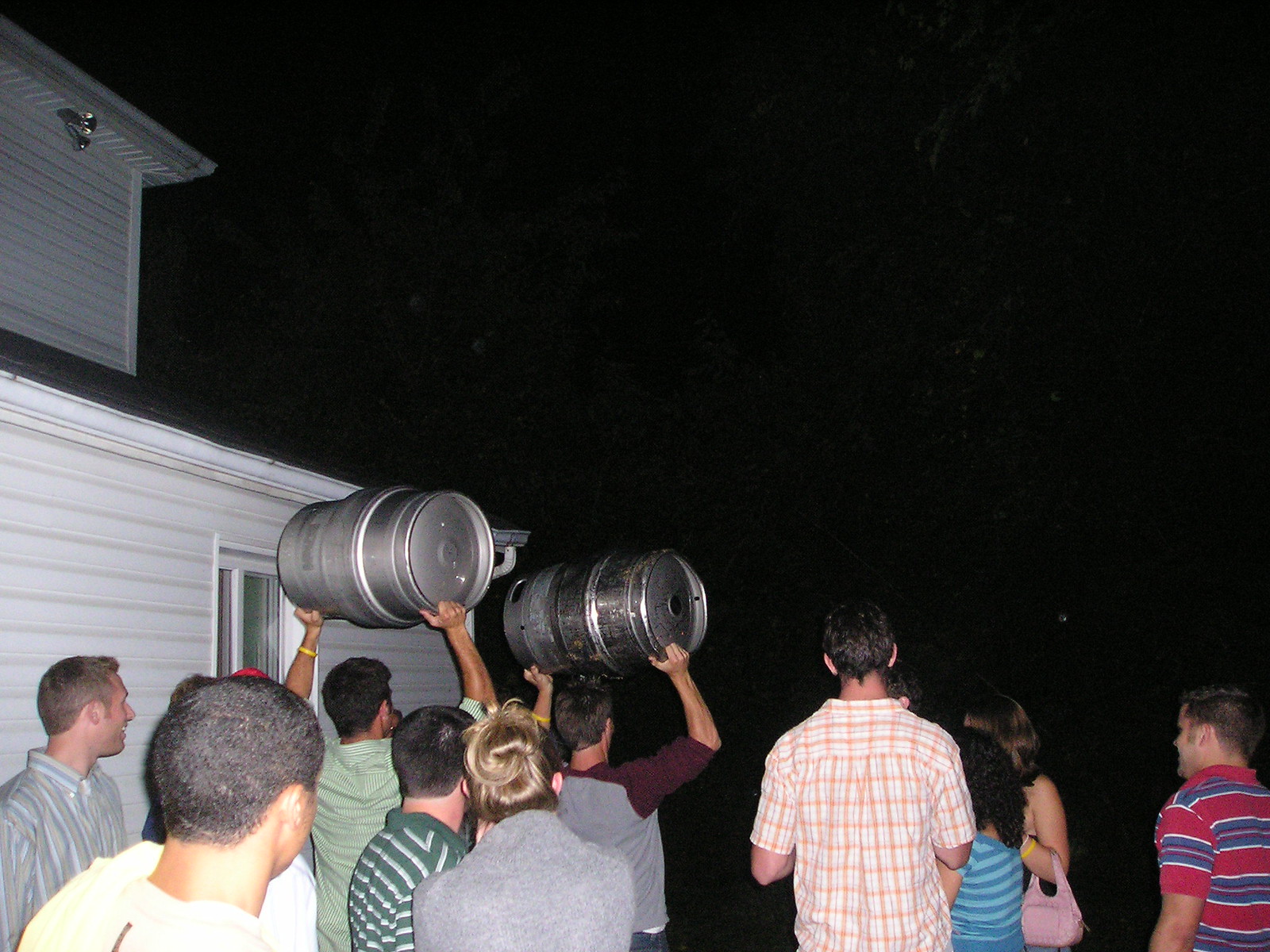In this nighttime outdoor scene, the sky is pitch black, and to the left side of the image, there's a partially visible two-storied house with white vinyl siding and a black roof. You can see a window on the house. In the foreground, around ten young people, possibly college or high school students, are gathered. Their backs are mostly shown, and they appear to be walking away from the camera. The group is predominantly male with a few females. Two young men, positioned in the middle left of the image, are prominently holding silver kegs above their heads. One of them is wearing a green shirt, while the other is dressed in a gray shirt with burgundy sleeves. Both young men have yellow wristbands on their left wrists. The group is uniformly looking in the same direction, possibly towards an event or party, into the dark night.